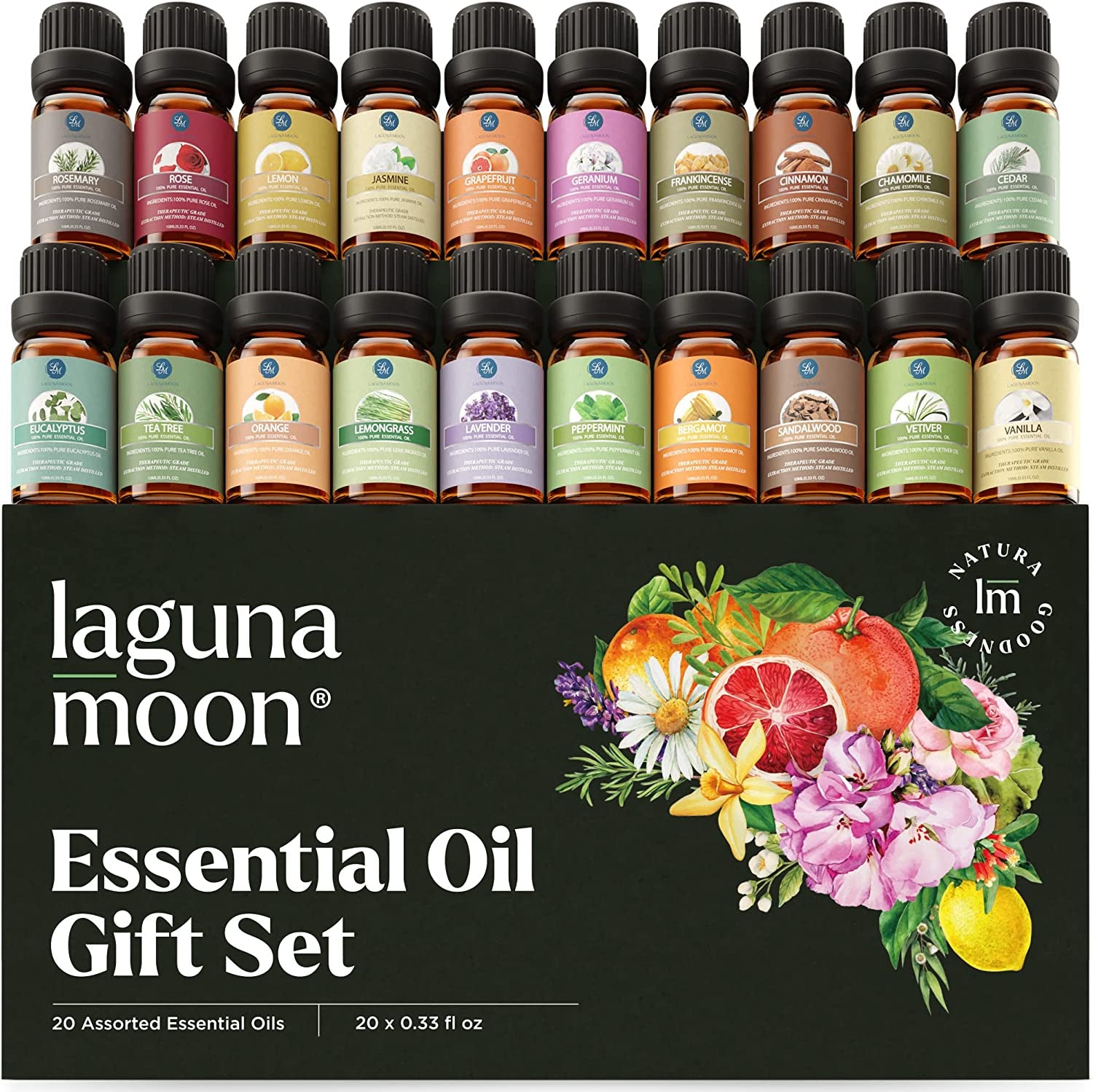This photograph showcases a Laguna Moon essential oil gift set, presented in a sleek black box with detailed white text. The bottom portion of the box features "Laguna Moon" in white lettering, followed by "Essential Oil Gift Set" in larger white letters, and further beneath, in smaller text, it specifies "20 assorted essential oils," each being 0.33 fluid ounces. Adjacent to this text, a vibrant illustration displays a variety of fruits, including grapefruit, oranges, and lemon, accompanied by pink, yellow, and white flowers with green leaves. The illustration also contains the phrase "Natura Goodness" with an "IM" integrated into the design.

The top section of the box showcases the 20 essential oils, neatly arranged in two rows of 10, each housed in clear bottles with black tops. The labels of these bottles are color-coded to represent their respective scents, adding a visually appealing array of colors. The oils included are rosemary, rose, lemon, jasmine, grapefruit, geranium, frankincense, cinnamon, chamomile, cedar, eucalyptus, tea tree, orange, lemongrass, lavender, peppermint, marjoram, sandalwood, vetiver, and vanilla. The thoughtful packaging design, combined with the vibrant labels and the diversity of included scents, makes this gift set both attractive and practical for essential oil enthusiasts.